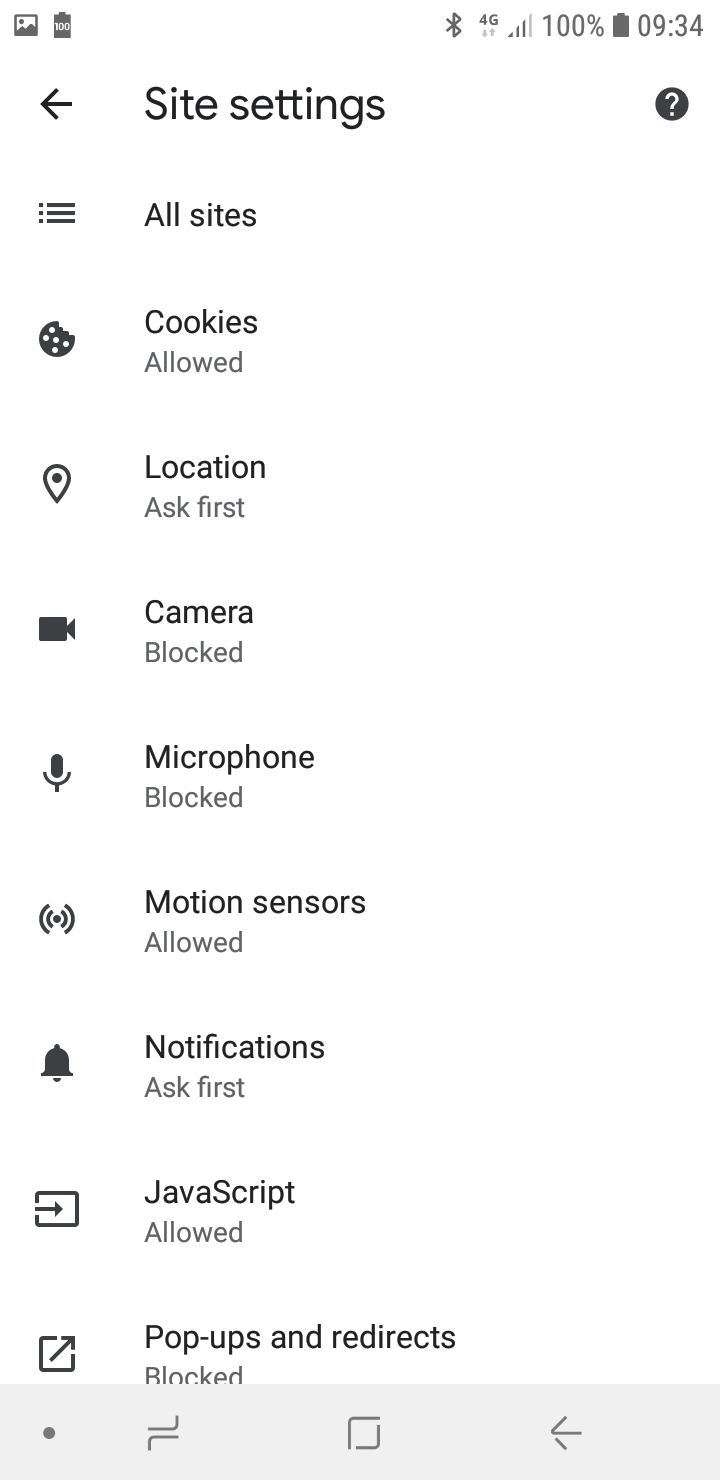The screenshot displays various settings and icons on a mobile device. At the top, the status bar shows "100% 0934," indicating full battery and the time as 9:34 AM. The signal strength is represented by 3 out of 4 bars, along with a Bluetooth icon. Below the status bar, there is a left-pointing arrow labeled "Site settings." Adjacent to this is a black circle featuring a white question mark. Below this section, a series of settings are listed:

1. A menu icon with three horizontal lines, labeled "All sites."
2. A cookie icon resembling a cookie, with the text "Cookies allowed."
3. A location pin icon, with the text "Location asked first."
4. A camera icon, labeled "Camera blocked."
5. A microphone icon, labeled "Microphone blocked."
6. The text "Motion sensor allowed."
7. A bell icon, with the text "Notification asked first."
8. A rectangle with a right-pointing arrow on its left, labeled "JavaScript allowed."
9. A square icon with a diagonal line through it, labeled "Pop-ups and redirects," followed by the text "Blocked."